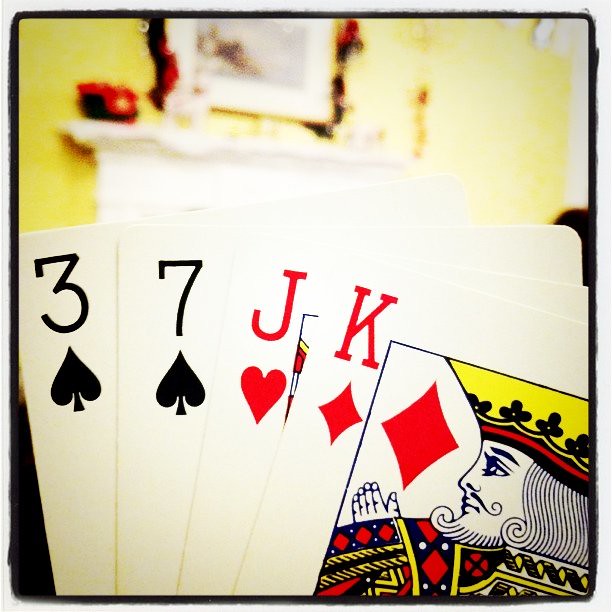In this image, a person is splaying out four playing cards against a visually intriguing background. The photo is framed with a black trim, with a blurred backdrop that gives context to the scene. The walls in the background are painted a soft yellow. Dominating the center of the image is a white fireplace, above which hangs a pitcher adorned with draping elements on its sides. The playing cards displayed in the foreground include the King of Diamonds, the Jack of Hearts, the Seven of Spades, and the Three of Spades. Notably, the King of Diamonds and the Jack of Hearts are red, while the Three and the Seven of Spades are black. On the mantle of the fireplace, a black pot is visible, seemingly holding vibrant red flowers with touches of yellow. To the top right of the image, the edge of a window sill can be discerned, adding a subtle architectural element. The right side of the background appears more blurred and obscured compared to the left, enhancing the focus on the cards.